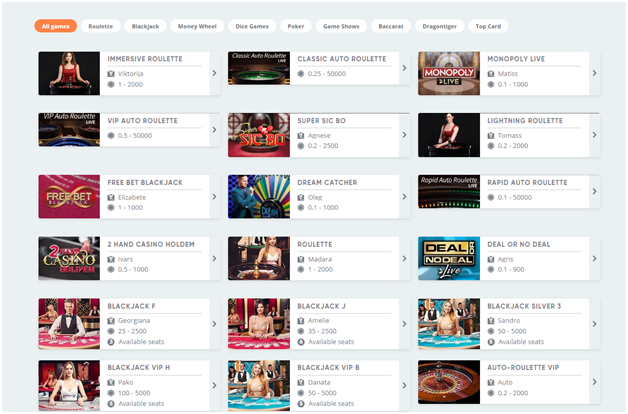The image showcases a webpage dedicated to online games, characterized by a clean, light gray background. At the top of the page, a navigation bar features a series of clickable buttons. The first button, labeled "All Games," is distinctively highlighted in orange with white text, while the subsequent buttons are white with black text and include the following options: Roulette, Blackjack, Money Wheel, Dice Games, Poker, Game Shows, Baccarat, Dragon Tiger, and Top Card.

Below this navigation bar, the page is organized into three columns, each containing a selection of interactive game thumbnails accompanied by brief descriptions and numerical details. Each game entry features a vivid image representative of the game itself, and to the right, within a rectangular box, the game's name and pertinent statistics are displayed.

In the first column, the games listed are:
1. Immersive Roulette
2. VIP Auto Roulette
3. Free Bet Blackjack
4. Two-Hand Casino Hold'em
5. Blackjack F
6. Blackjack VIP H

The same layout and organization continue in the second and third columns, each housing six games. This structured and detailed design ensures easy navigation and access to a variety of online gaming options available on the website.